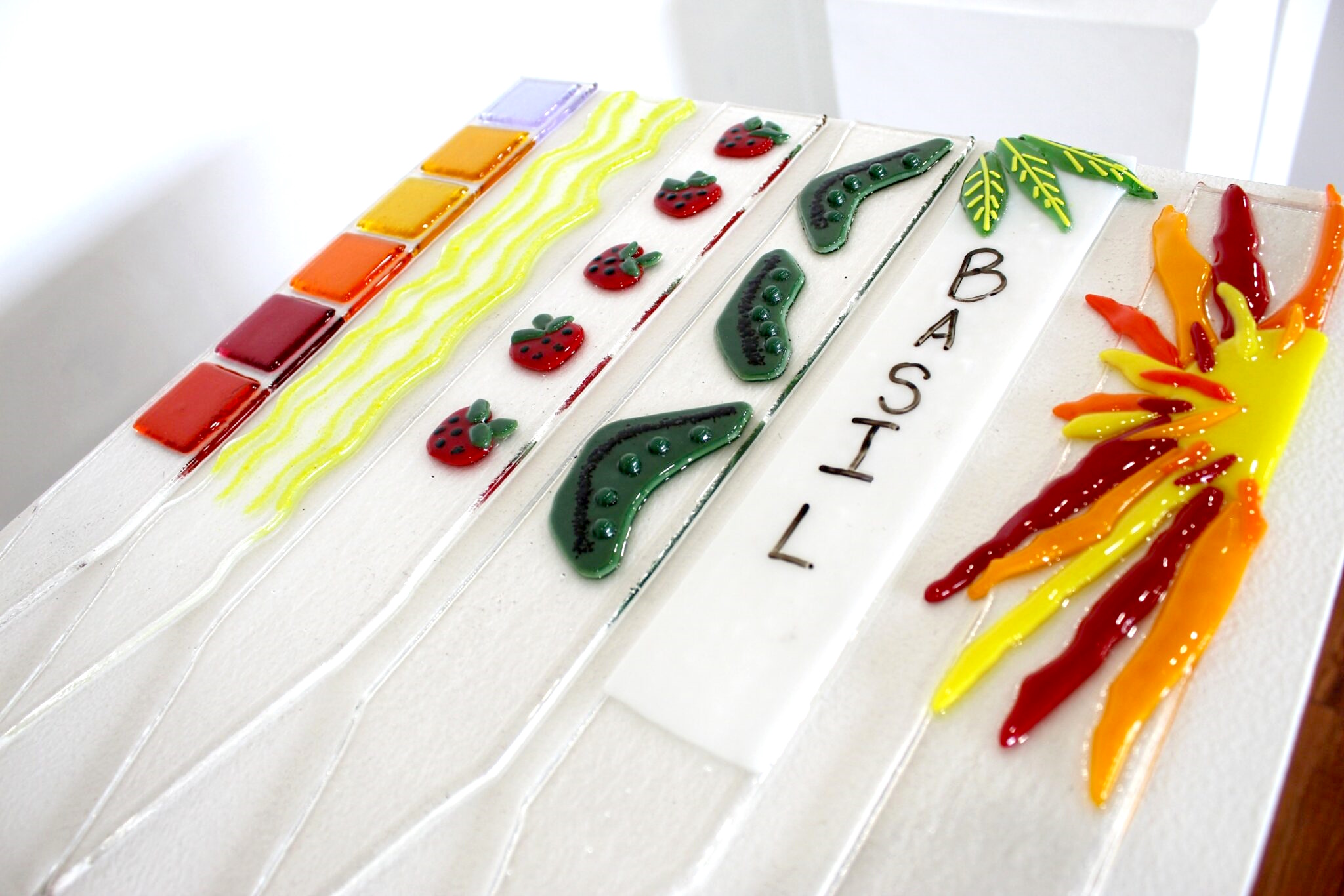In this image, there is an intricate and colorful piece of artwork showcased against a plain white background. The artwork is arranged on individual white planks connected together, forming a series of visual elements. At the forefront, the word "BASIL" is prominently displayed along one side. The composition features an array of strawberries, half of a sun with vivid hues of yellow, orange, and red, and green boomerang shapes. There are also multiple squiggly lines of yellow paint contributing to the vivid scene. The artwork has elements that resemble peas in a pod and various color transitions from deep red to clear yellow. Its orderly yet artistic arrangement suggests it could be a decorative piece for a refrigerator or table design, though its exact purpose remains ambiguous. The overall effect is lively and vibrant, showcasing a skillful blend of colors and shapes, culminating in a unique visual experience.